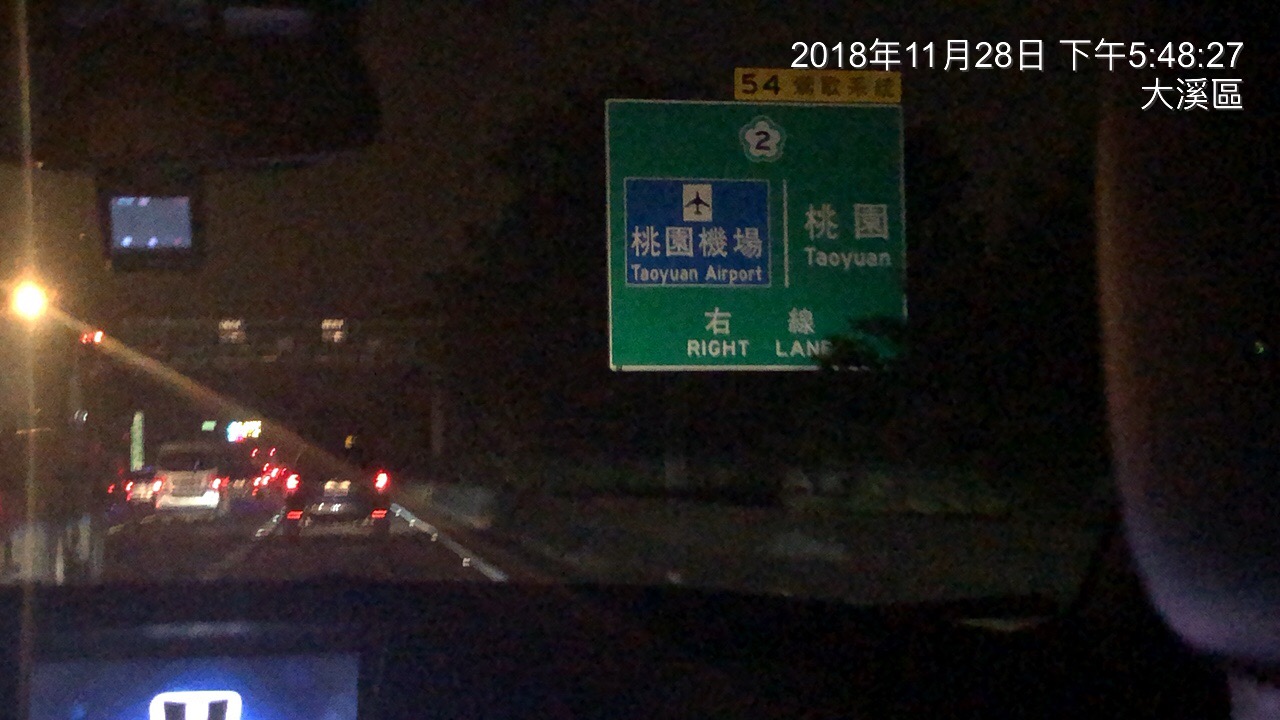This landscape-oriented photograph, taken from the passenger seat of a moving car on the freeway, captures a typical scene of early evening traffic. In the upper left corner, the outline of the rear view mirror is visible, anchoring the perspective from within the vehicle. Up ahead, several cars are pressing on their brakes, creating a sequence of glowing red taillights that stand out against the dimming light. Towards the middle-right of the image, a billboard in a foreign language is present, prominently displaying a road sign in shades of green, blue, and yellow. In the top right corner, a date and time stamp read "11-28-2016 5:48," marking the precise moment this snapshot was captured.